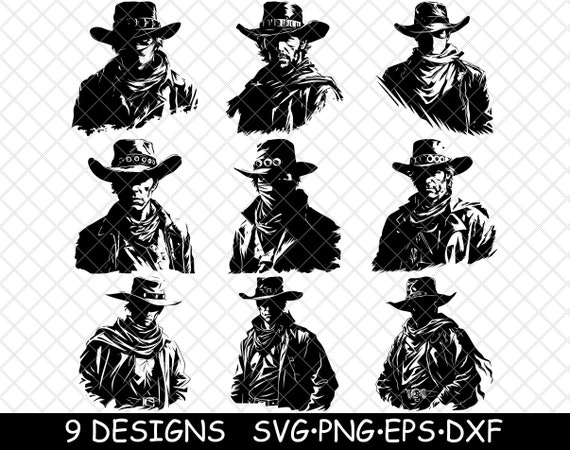The image is a black-and-white sketch featuring nine cowboy-like figures from the 19th century, each donning traditional cowboy hats and scarves around their necks or faces, evoking the rugged persona of Wild West bandits. The figures are organized in three rows of three, with those at the top depicted from the shoulders up, while the rest are shown from the waist up. The background is a plain white, overlaid with a subtle gray crosshatch pattern reminiscent of a chain-link fence. At the bottom of the image, a black horizontal band contains white text reading "9 designs • SVG • PNG • EPS • DXF" in all capitals.